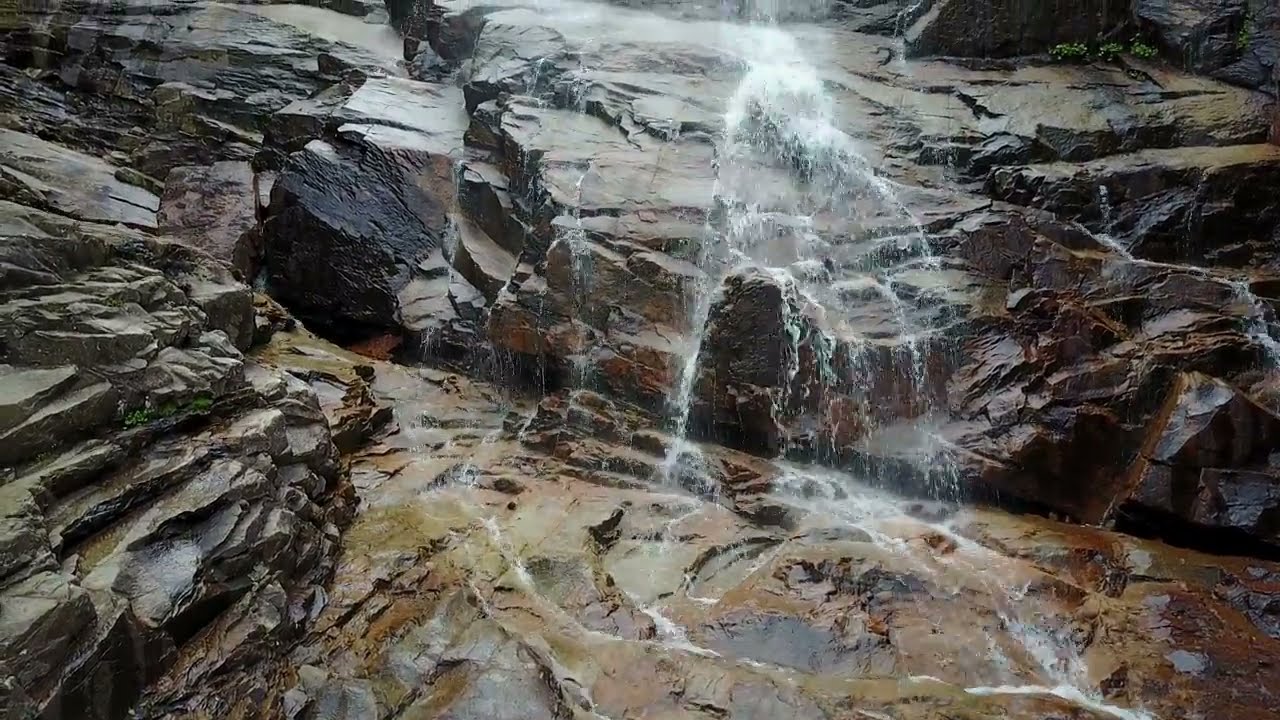The photograph captures a modest waterfall cascading down a rocky mountain face, taken from a vantage point at the bottom looking upward. The water, although not thick, flows steadily and separates as it interacts with the rocky layers, creating a visually appealing white water effect. The rocks themselves are predominantly gray, with parts shaded in dark brown, orange, and tinged green from moss. The face of the mountain is stratified, with many layers and crevices that appear to have formed naturally over time. Sparse plants peek through the crevices where they can, adding a touch of life to the otherwise barren stone. The combination of these rugged, varied hues and textures, accented by the cascading water, creates a scene of understated beauty.